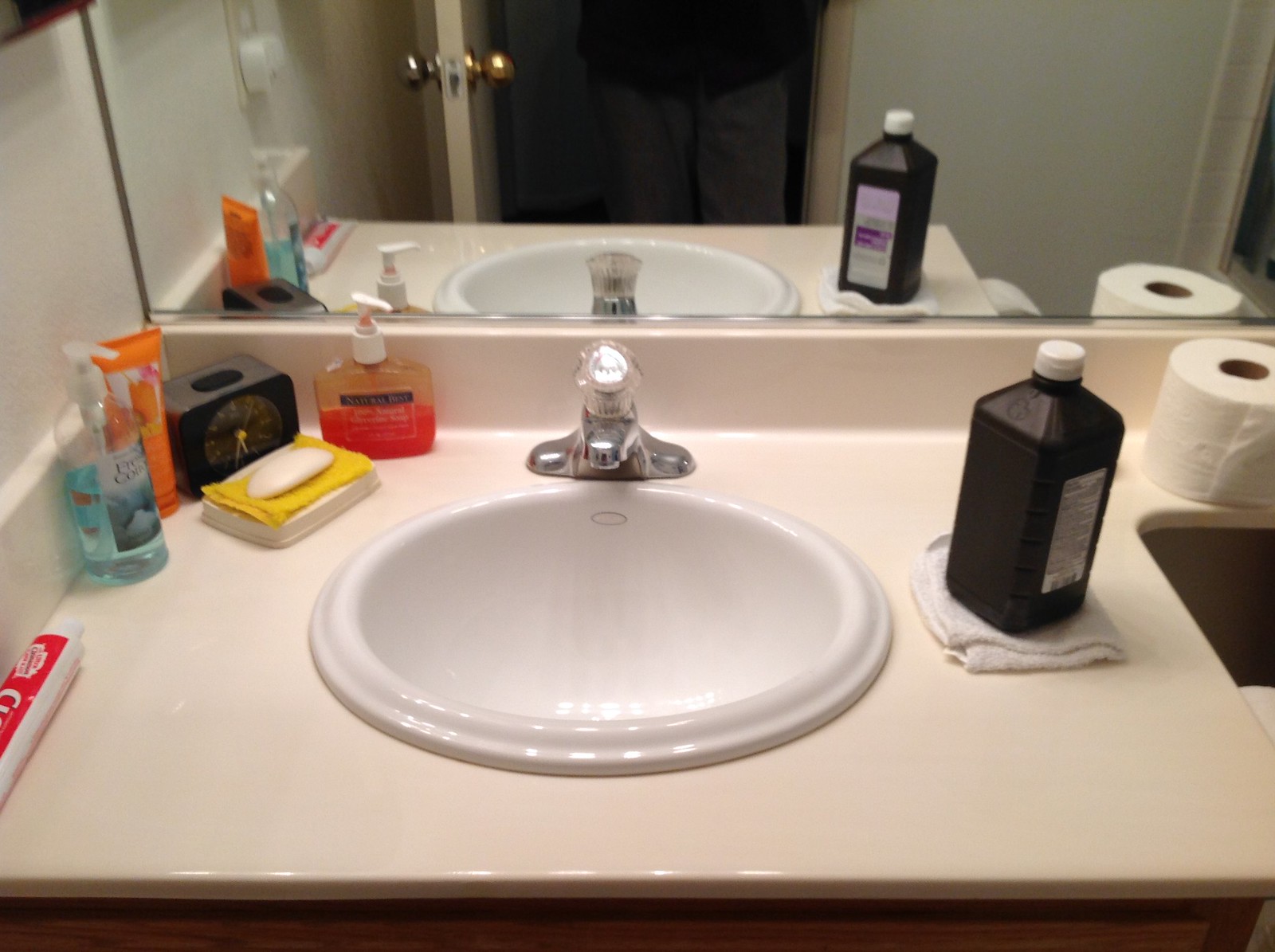This image captures a bathroom scene viewed directly facing the sink area, with a slight downward angle as if from the mirror's perspective. The sink rests on a smooth, light beige off-white countertop that is unadorned with any patterns or textures. To the far right of this countertop is an open cavity, revealing a faint glimpse of something white below, though the exact details remain unclear. Just above this opening, a roll of toilet paper is perched.

To the immediate right of the sink sits a neatly folded white washcloth topped by a bottle, likely containing hydrogen peroxide. Positioned in the rear right corner, a pump bottle of liquid soap stands ready for use, complemented by a bar of soap resting on a yellow washcloth.

An adjacent clock with a brown base, featuring an oval opening at the top, provides the time. Nearby items include another bottle, possibly hand sanitizer, an orange container, and a tube that might be toothpaste, all nestled in the corner of the countertop.

A rectangular mirror prominently dominates the background, reflecting the open bathroom door. Through the doorway, a person wearing a dark shirt and possibly gray pants is visible, adding a human element to the serene setting.